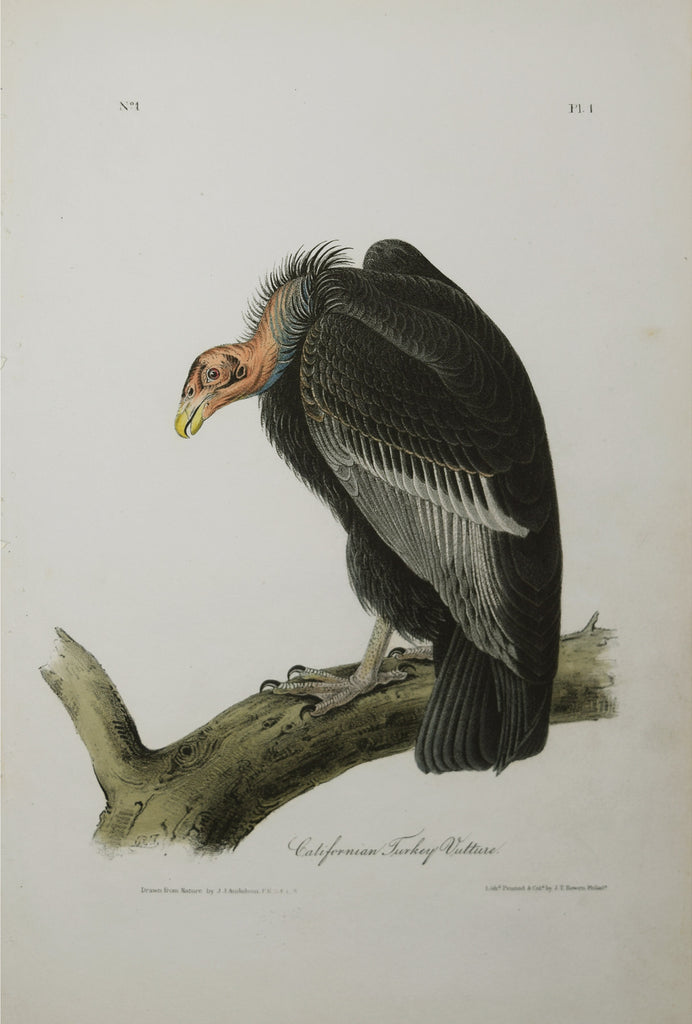In this color detail illustration on a light gray piece of paper, a Californian turkey vulture is prominently perched on a thick tree branch that spans diagonally from the bottom left to the upper right of the image. The branch appears to be a mix of green, black, and light brownish gray hues, capturing a realistic texture. The vulture, with its whitish gray talons gripping the branch, has its body mostly facing the right side of the image. Covered in long, black feathers with distinctive white tips on the wings, the vulture's head is tucked downwards. The bird has a striking orange head and neck, which is somewhat bald with thin, fur-like feathers at the base, and it features a sharp yellow beak. The bird's eyes seem to peer out towards the viewer despite the downward positioning of its head. The illustration is framed within a rectangular format that is taller than it is wide, with darker shading towards the bottom of the image. Encircling the bird, small, partially legible text identifies the species as a Californian turkey vulture.